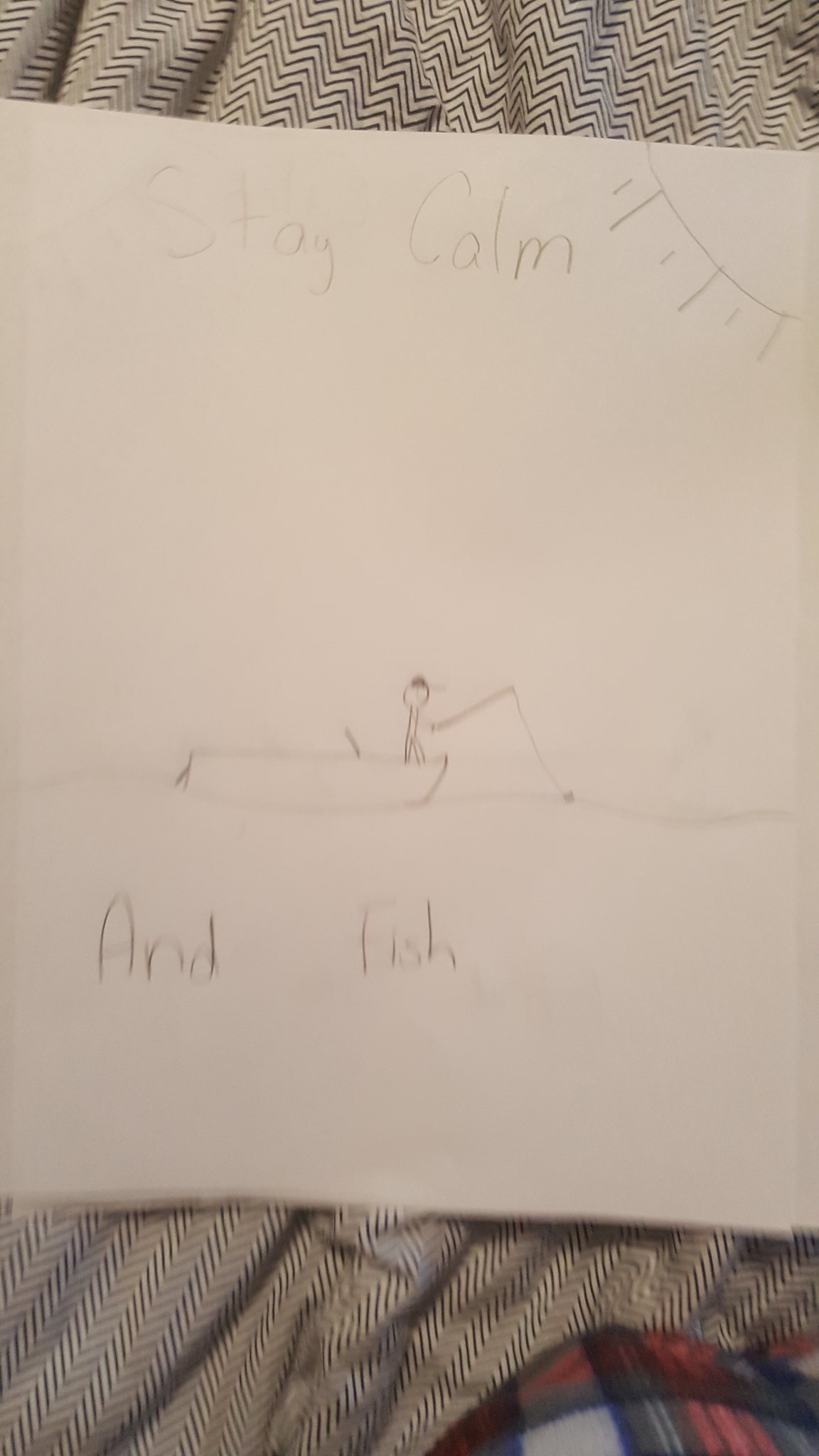This detailed image depicts a child-like drawing on a sheet of white paper, captured in a portrait format. The image, about three to four times taller than it is wide, shows a simplistic pencil drawing that spans across a piece of landscape-oriented paper, which is too large to fit entirely within the frame, cutting off the left and right edges. The top of the paper bears the hand-written message "stay calm" in what appears to be a child’s handwriting. Just beneath this, in the upper right corner, a partial sun is illustrated with alternating long and short rays emanating from its curve.

Midway through the image, a wavy line represents water, stretching across the paper. Above this line, there is a rudimentary drawing of a rectangular boat, with a stick figure standing in front of it. The stick figure, characterized by a round head, a baseball cap, and simplistic limb lines, holds a fishing pole. The pole is drawn as a darker, straight line angled upward with a thinner line extending downward into the water, ending in a small circle, suggesting a fishing hook. Below the waterline, the words “and fish” are written, completing the calming message.

The background of the image includes a soft-looking, bunched-up blanket or fabric with jagged black and white stripes at the top and bottom, taking up roughly the top 10% and bottom 20% of the image. Additionally, there is a section of plaid fabric in the bottom right-hand corner, displaying a pattern in blue, gray, white, and red. The overall scene combines the innocent simplicity of a child's drawing with the comforting textures of the surrounding fabrics.